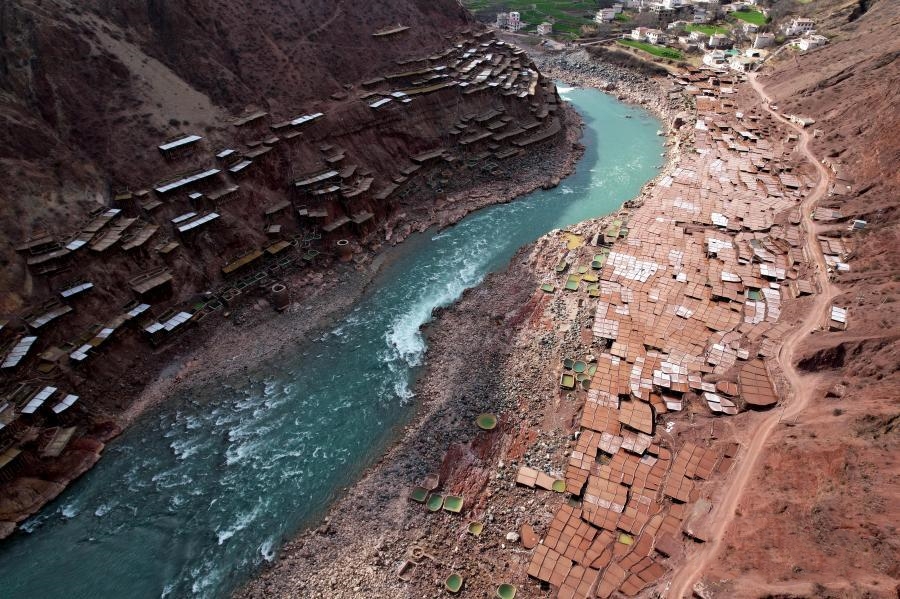The photograph captures a striking canyon scene with a clear, blue river running through its center. Red clay dirt frames the canyon, and along its sides and base, clusters of structures, possibly houses or trailers, are prominently visible. Some of these structures are built directly into the cliff walls on the right-hand side, characterized by white walls and beige or tan-red roofs. There is a dirt road running along the right-hand base of the canyon, but no visible access on the left, raising questions about connectivity for the buildings there. Towards the end of the canyon, near a bend in the river, there are more houses surrounded by vivid green grass. The foreground and the initial stretch along the river feature an expanse of mud, which may be clay in varying stages of drying, lending a patchwork of textures and colors to the landscape. The presence of round green pails suggests some form of activity, perhaps related to clay or tile production. Despite the vivid natural and built environment, the image is devoid of people, adding to its serene, almost timeless quality.